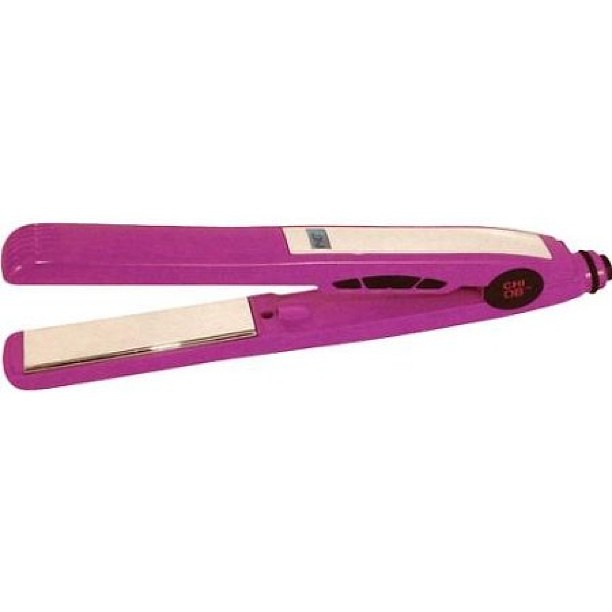This image features a retro-looking hair straightener, prominently centered against a totally white background. The hair straightener itself is a light lavender purple with significant white and black detailing. It has two levers that meet in the middle, designed to close and straighten hair. Each lever features a white panel where the hair would be placed, bordered by a slim strip of silver metal. On the top lever, there's an additional white rectangle near which three black, fan-like grooves are visible. At the junction where the levers meet, there is a distinctive black dot. You can also notice a black circle on one side with red lettering that appears to read "C-H-I-O-B," possibly indicating the brand. The overall design and aesthetic suggest a vintage or older style of hair straightener. The device also includes a digital display on the top portion, likely for temperature readout.